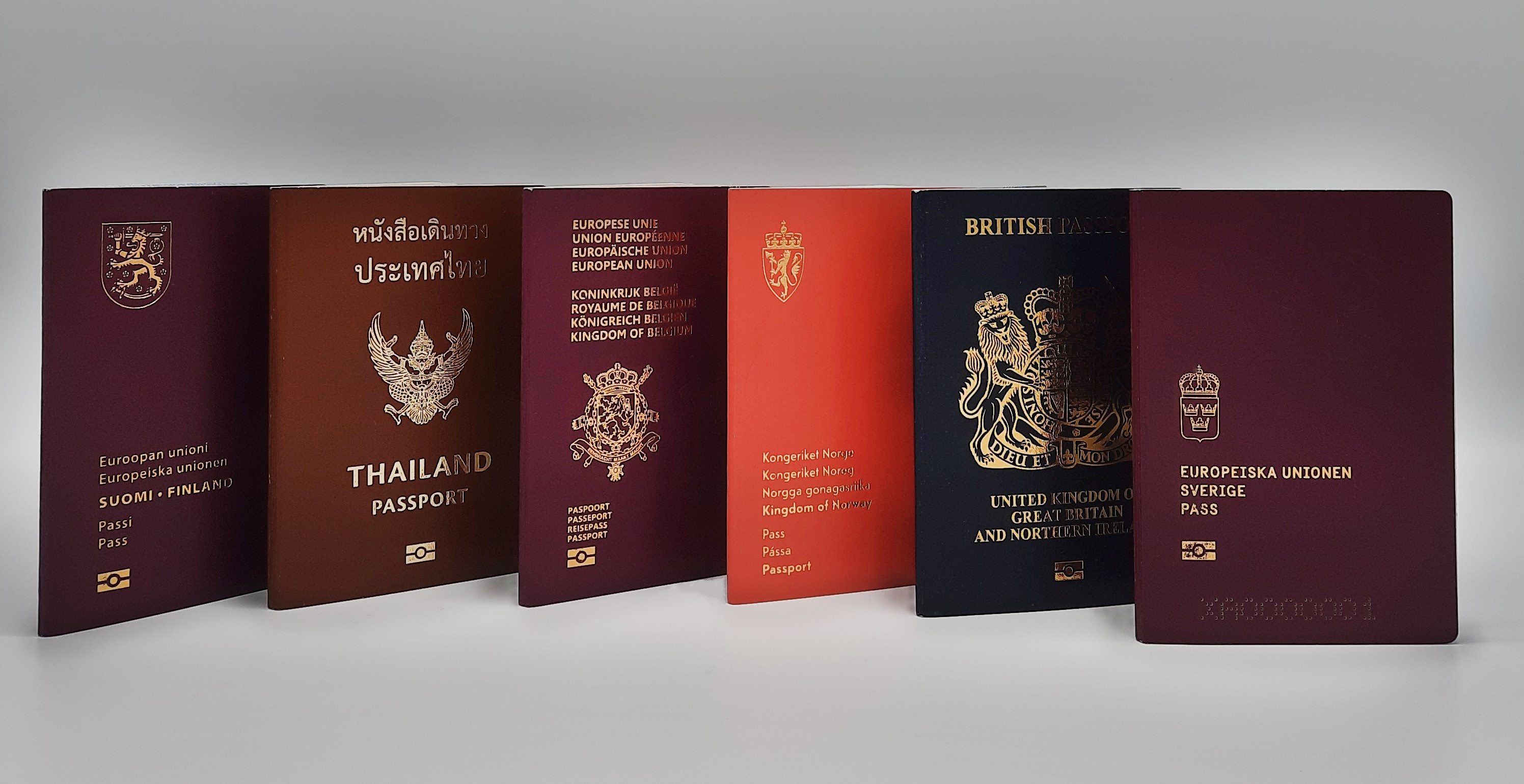The image displays six passports arranged in a row from left to right, standing upright against a light bluish-gray background. Each passport features distinctive colors and gold text with various national emblems and insignias. The first passport on the far left is maroon and displays the Finnish coat of arms along with "Suomi Finland Passport" inscribed in gold. Next, there is a brown passport with a gold emblem featuring a native bird, labeled "Thailand Passport." The third passport, also maroon, is marked with "European Union" and a gold shield symbolizing its European origin. In the middle, a red passport showcases the Kingdom of Norway’s shield at the upper left, outlined in gold. To the right, a navy blue passport bears the British coat of arms with the word "British" prominently visible at the top. The last passport on the far right is another maroon document, marked with "Europeiska Union," accompanied by a gold crown icon, signifying its European context. The passports, diverse in origin and design, are unified by their elegant gold detailing and the consistent arrangement on the neutral background.